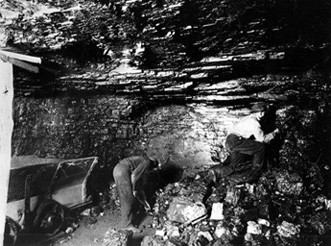This is a small, very old black and white photograph depicting a scene within a coal mine. The image shows a cavernous space where the ceiling and walls are made of the same rocky material, creating a claustrophobic atmosphere. In the lower left corner, mining equipment is visible alongside a man in a uniform, who is hunched over and perhaps shoveling coal into a nearby tram or carriage. This tram has a visible wheel and compartments for transporting materials. Another man appears to be climbing or sitting near the rocky wall, wearing what seems to be a hard hat with a lamp on the front, though the details are a bit unclear due to the photo's small size. A large pile of rocky debris or coal is on the right side of the image, contributing to the impression of active labor. The ceiling, while rocky and uneven, is tall enough to accommodate the standing man but might be around ten feet high. The overall scene is devoid of any caption or writing, enhancing the historical and timeless aspect of this black and white snapshot of life in a coal mine.